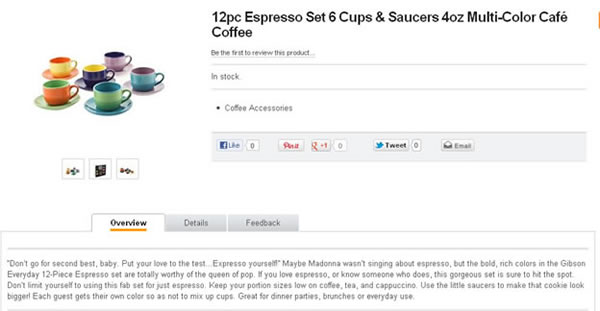A detailed webpage displays a vibrant 12-piece espresso set, which includes 6 cups and matching saucers, each holding 4 oz of coffee. The set is available in an array of multicolored options—orange, yellow, green, blue, purple, and another shade of yellow. Above the set, text prompts customers to 'Be the first to review this product,' highlighting its availability as 'In Stock' and categorizing it under 'Coffee Accessories.'

On the left side of the page, images showcase the colorful cup and saucer sets, with the current image selected out of three available options. Social media buttons for Facebook, Pinterest, Google, Twitter, and an email link are conveniently positioned for easy sharing.

At the bottom of the webpage, three tabs organize information under 'Overview,' 'Details,' and 'Feedback.' The overview playfully encourages espresso enthusiasts to choose this vibrant set, evoking the iconic flair of the queen of pop with the statement: 'Don’t go for the second best baby, put your love to the test. Espresso yourself.' While the text hints that the referenced song lyrics might not be about espresso, it underscores the set's bold, rich colors by Gibson Everyday as truly fit for coffee lovers.